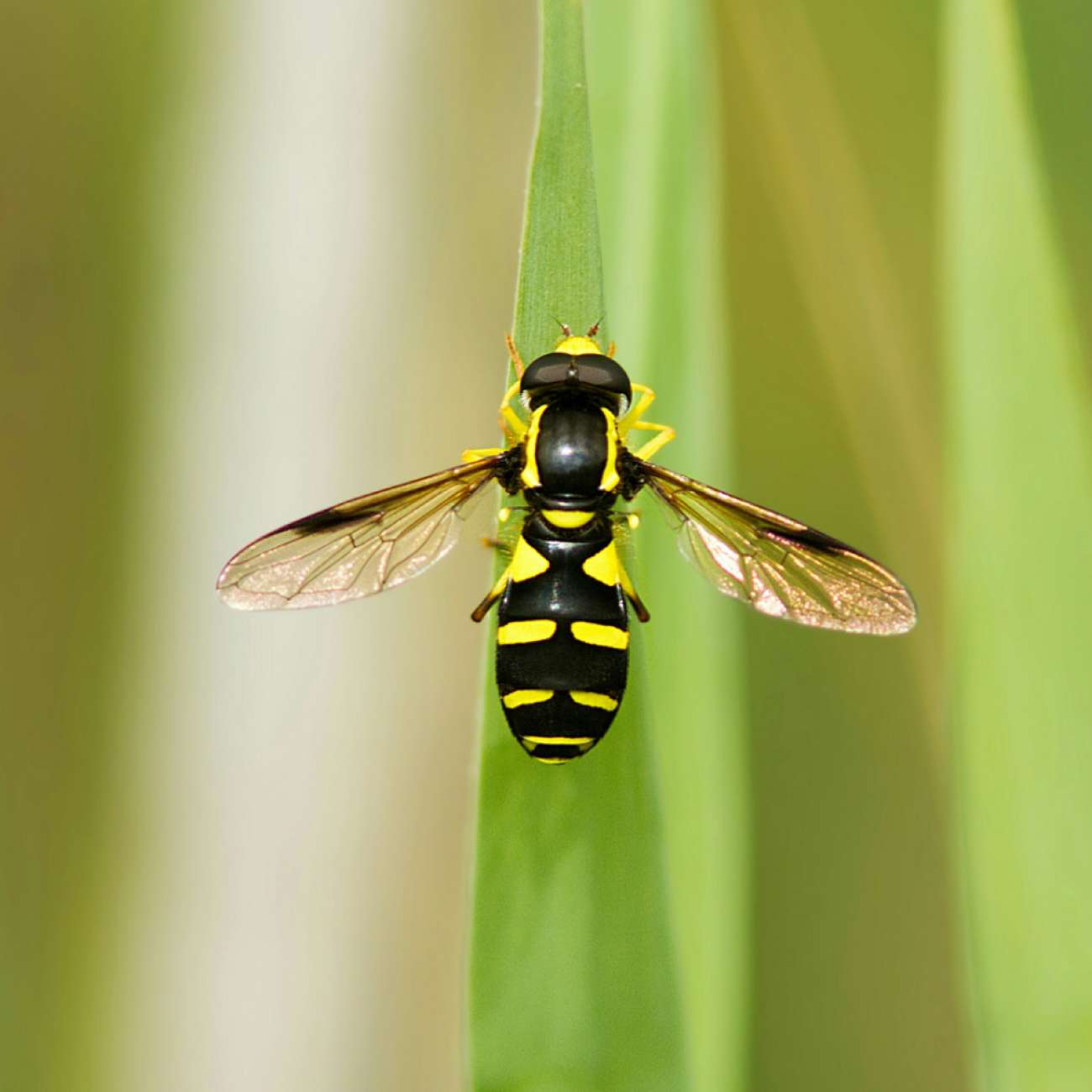This detailed close-up image captures a bee or wasp perched vertically on a blade of grass, appearing almost like a meticulously crafted model. The insect, about the width of the grass blade, has elegantly outstretched wings that seem nearly transparent, resembling acrylic or glass. Its black abdomen, adorned with vibrant yellow stripes and subtle yellow markings, gleams under the natural light, giving its glossy surface a smooth appearance. The insect's legs also bear yellow accents, and its arms grasp firmly onto the top portion of the grass blade. In the backdrop, a series of additional blades of grass appear blurred, emphasizing the sharp focus on the bee or wasp. This composition, with its lifelike yet almost figurine-like representation, combines elements of nature's simplicity with the detailed intricacy of a handcrafted model.